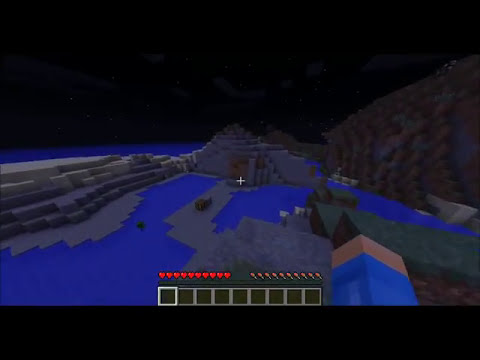The screenshot from the video game Minecraft showcases a first-person perspective at nighttime, characterized by a dark sky with white dots representing stars and subtle cloud formations. The scene is dominated by hues of blue and black. At the bottom center, there is an item selection bar with various icons, above which are red heart-shaped icons indicating the player's health and nearby food icons in red, brown, and white. The player’s blocky arm with a blue sleeve and peachy hand is visible on the right-hand side. The landscape is distinctly blocky, featuring gray stone mountains, a tall brown hill covered in green and brown grass-colored blocks, and a stone pathway leading to a crafting bench and a furnace in the center. The overall setting suggests the player is preparing for an adventure or engaging in resource gathering.